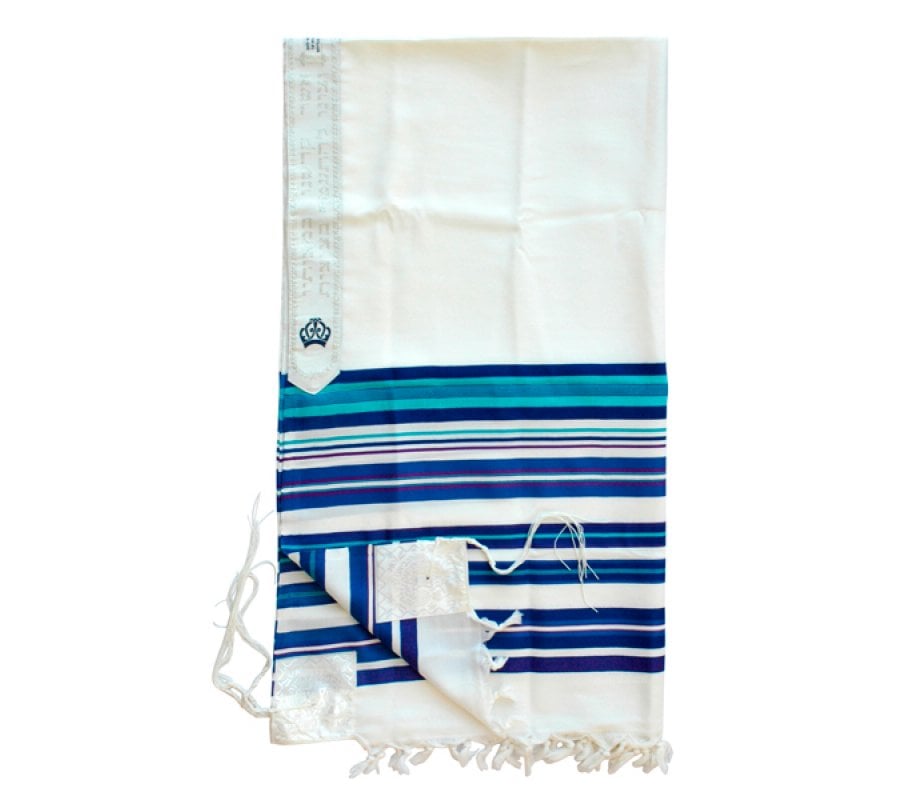The photograph captures a close-up image of a folded hand towel, set against a purely white background that eliminates visible edges. The towel is folded into a neat rectangular shape, with a fringe along one edge that is slightly frayed, hinting at its age and use. Predominantly white, the lower half of the towel features horizontal stripes in varying shades of blue, including navy, teal, dark, and light blue. These stripes alternate in random patterns down the towel. Notably, the bottom left-hand corner is turned up, forming a small triangle. Additionally, a sewn-on cloth label adorned with a crown is visible along the left-hand side, distinguishing the towel with its unique detail.